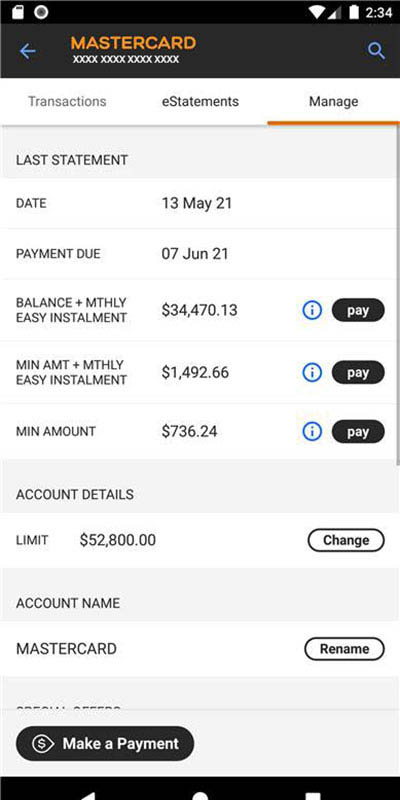The screenshot captures the interface of a MasterCard account management page viewed on a cell phone. In the top right corner of the screen, the current time (2:34) and a battery symbol are visible, accompanied by a black or gray status bar at the top. Below this bar, "MasterCard" is prominently displayed in orange, followed by a series of Xs representing a masked MasterCard number. 

Near the upper right, there's a "Manage" button, which appears to have been clicked to reveal the cardholder's detailed MasterCard information. The information includes:

- Last statement date: 13 May 2021
- Payment due date: 07 June 2021
- Balance plus monthly easy installment: $34,470.13

To the right of this section is a dark-colored oval button labeled "Pay" in white text.

Further down, the minimum amount plus monthly easy installment is shown as $1,492.66, accompanied by another "Pay" button. Below this, the minimum amount by itself is listed, again with a corresponding "Pay" button for payment options.

Additional account details include the account's credit limit, set at $52,800, along with a "Change" button. The account name is simply "MasterCard," with an adjacent "Rename" button appearing on the right side.

At the bottom of the screen, a large black oval button marked "Make a Payment" offers another option to initiate a payment transaction.